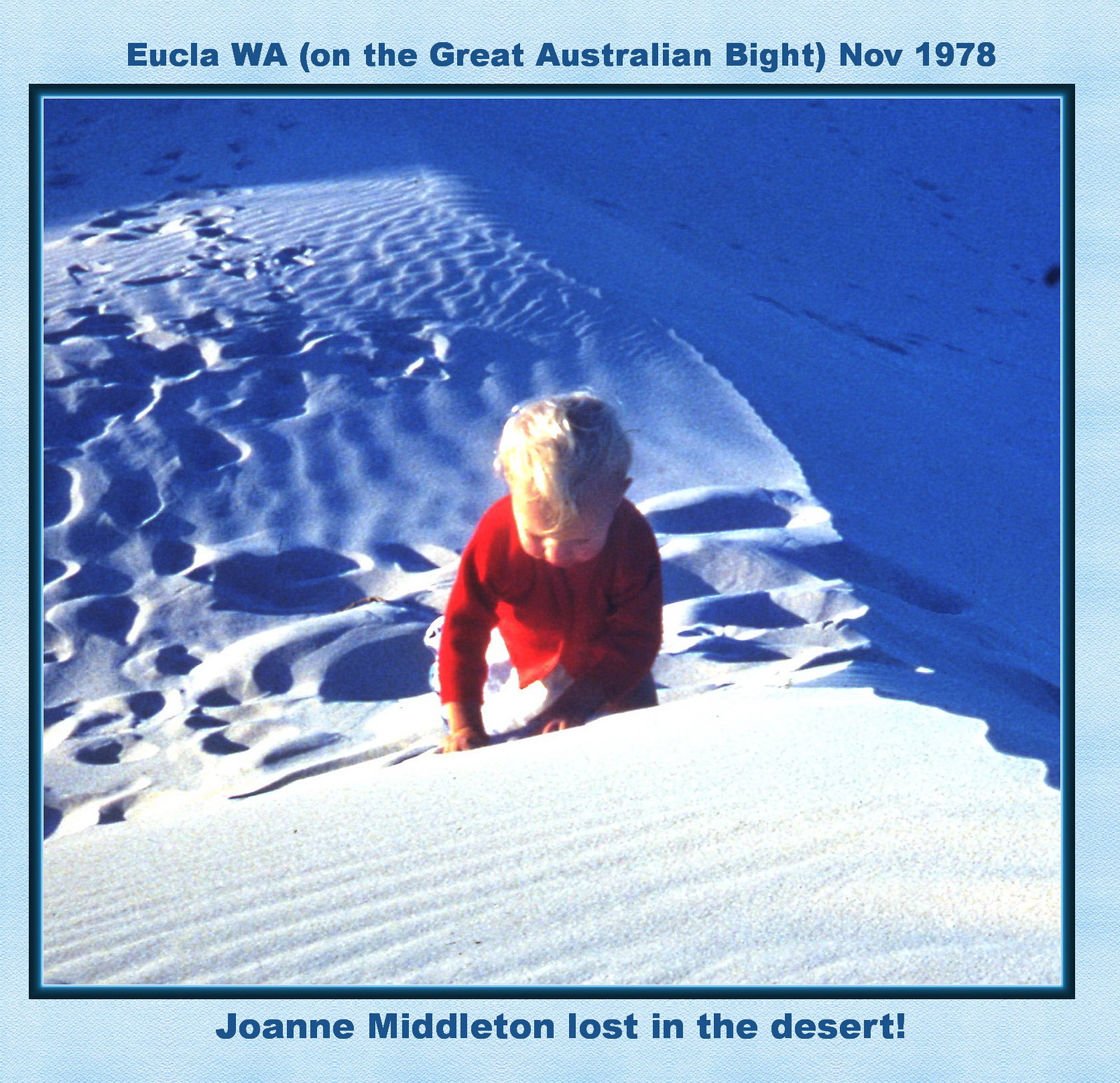The image is a vintage photograph framed with a light blue border and features blue font text at the top that reads, "Eucla, WA (On the Great Australian Bight), November 1978." Along the bottom, it says, "Joanne Middleton lost in the desert!" The photograph depicts a small child, around three years old, with curly blonde hair and fair skin, wearing a red long sleeve sweater and no gloves. The child is playing on a hill that appears to be covered in bright white sand but could be mistaken for snow due to its color and the lighting in the picture. Footprints are visible in the sand/snow, indicating that people have walked by. The setting is isolated, with no structures in sight, giving the impression of a desolate dune or hill. The child's face is mostly obscured as they look down while engaging with the ground.